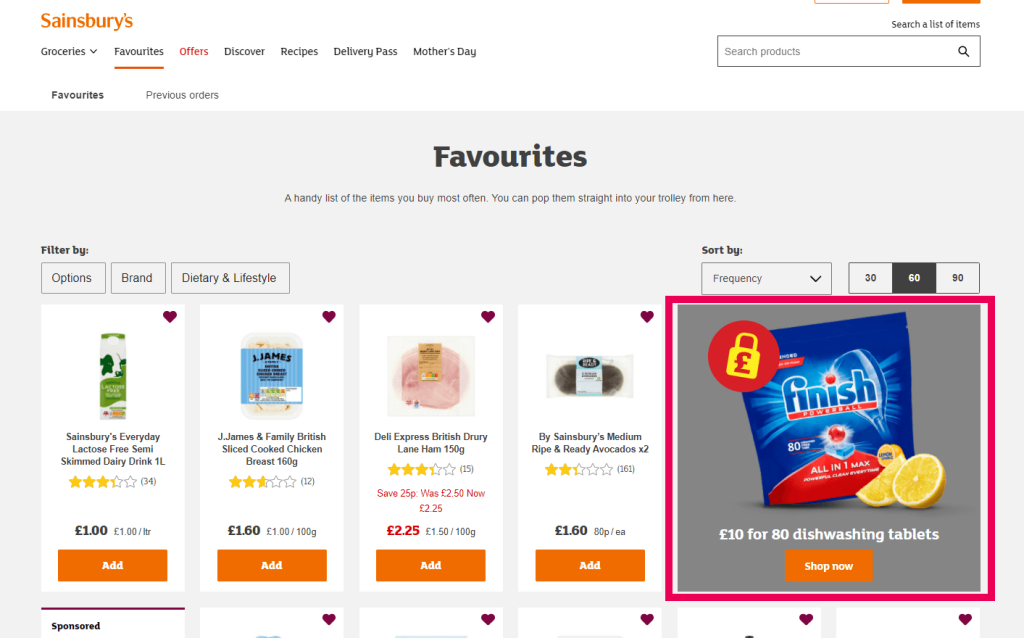The image is a screenshot of a webpage from the Sainsbury's grocery store website. The background of the page is white, featuring a light orange Sainsbury's logo at the top left corner. Below the logo is a horizontal navigation menu with the following tabs: Groceries, Favorites, Offers, Discover, Recipe, Delivery Pass, and Mother's Day. The tab titled 'Favorites' is highlighted in orange, while 'Offers' is marked in red. The remaining tabs are displayed in black text.

At the top right of the webpage is a white search bar bordered in gray, labeled "Search products" with a magnifying glass icon beside it. As you scroll down the page, the heading "Favorites" is displayed prominently in black text, with a subheading explaining that it is a handy list of items you buy most often and can be added directly to your cart from this page.

Beneath the heading are various grocery items. The page features filter options for 'Brand, Dietary, and Lifestyle' choices. Some of the food items displayed include:

1. A dairy milk drink, distinguishable by its white and green packaging with a cow illustration.
2. Cooked chicken breast from James and Family, displaying a blue logo.
3. Ham available for purchase.
4. Medium ripe and ready avocados.

Each item is accompanied by star ratings and an orange "Add" button in white text for adding the item to the cart.

On the right side of the page, there's a 'Sort By' section with options to display 30, 60, or 90 items per page, with the '60' option highlighted.

Below this section is an advertisement for Finish All-in-One Max Powerball dish detergent. The product is presented in a dark blue bag with the Finish logo in blue. The packaging is opened, revealing the contents next to a lemon wedge. The product description mentions it's priced at 10 pounds for 80 dishwashing tablets. An orange "Shop Now" button in white text is available below the product details.